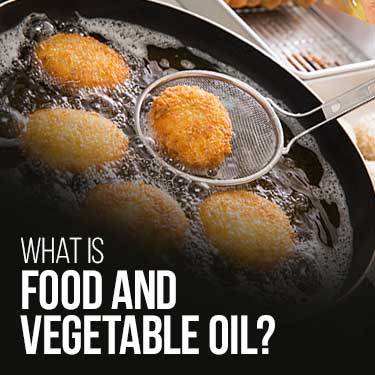The image depicts a black frying pan sitting on a stove, filled with bubbling vegetable oil. Inside the oil, there are several circular, golden-brown, crispy items that resemble either little cakes or chicken nuggets. The oil is foaming with white bubbles. Out of the five pieces in the oil, four are floating while one is being lifted out with a black spoon strainer to drain off the excess oil. At the bottom left corner of the image, white text reads, "What is food in vegetable oil?" At the top right corner, there is a silver tray containing some brown food items which resemble hot dogs, and it appears to be a holding or draining vent area. The scene appears to be a cooking process, possibly in a kitchen.